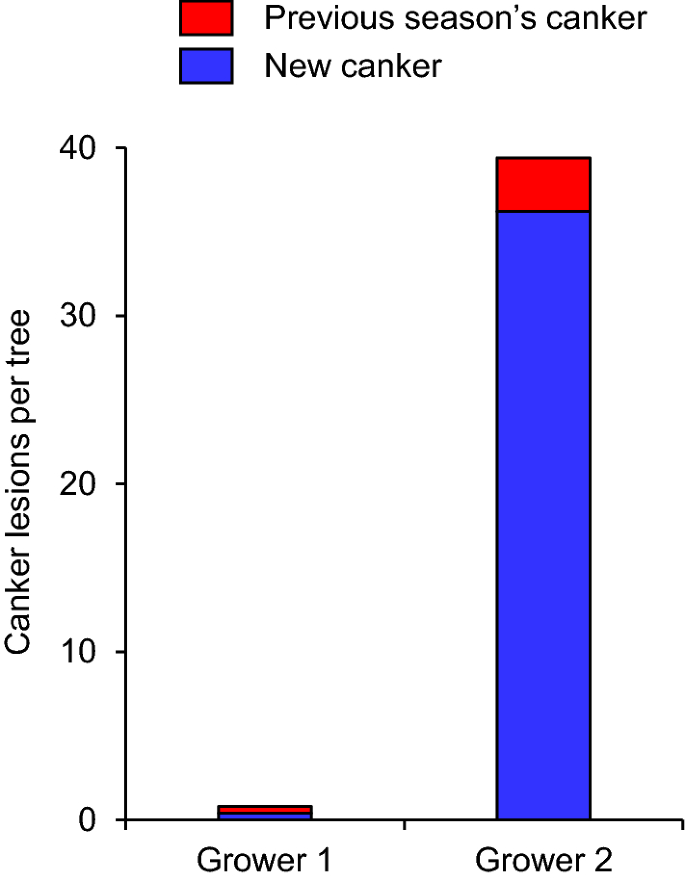The image depicts a detailed bar graph comparing canker lesions per tree between two growers across two seasons. The vertical axis, labeled "Canker Lesions per Tree," ranges from 0 to 40 in increments of 10. The horizontal axis categorizes the data by "Grower 1" and "Grower 2." 

Each grower is represented by two bars: a red bar for the previous season's cankers and a blue bar for the new season's cankers. The key at the top of the graph clarifies that red signifies "Previous Season's Canker" and blue denotes "New Canker." 

For Grower 1, the graph shows minimal infection, with the red and blue bars barely reaching the value of 1. Conversely, Grower 2's red bar, indicating past infections, reaches approximately 4, while the blue bar drastically increases to just over 35, illustrating a significant surge in new canker lesions per tree in the current season. This stark contrast highlights a severe increase in canker infection for Grower 2 compared to the prior season, drawing attention to the substantial impact of the new infection.